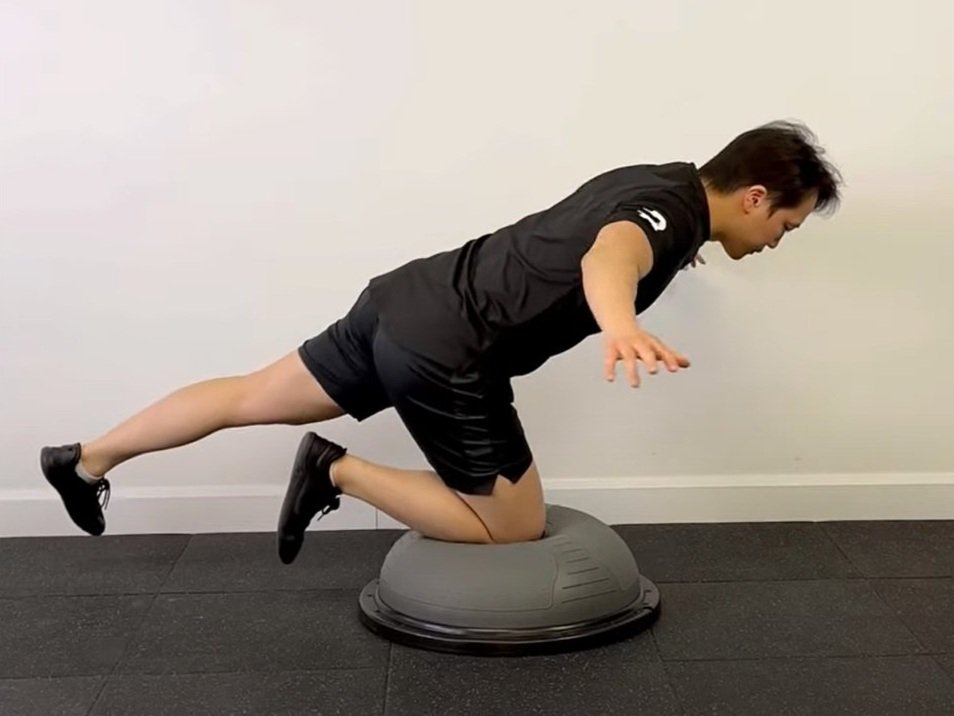In this photograph, an Asian man with short black hair, possibly in his thirties, is performing an exercise indoors against a white or cream-colored wall on a black padded floor. The man is seen in profile, balancing on a gray half-ball exercise equipment with his right knee. His body is angled diagonally at about 45 degrees to the ground, maintaining balance with both arms extended out to the sides. His left leg is stretched out straight behind him. The man is dressed in black athletic attire, including a t-shirt, shorts, and shoes. The detailed posture and use of the half-ball suggest this might be part of a demonstration or tutorial aimed at showcasing this balancing exercise.